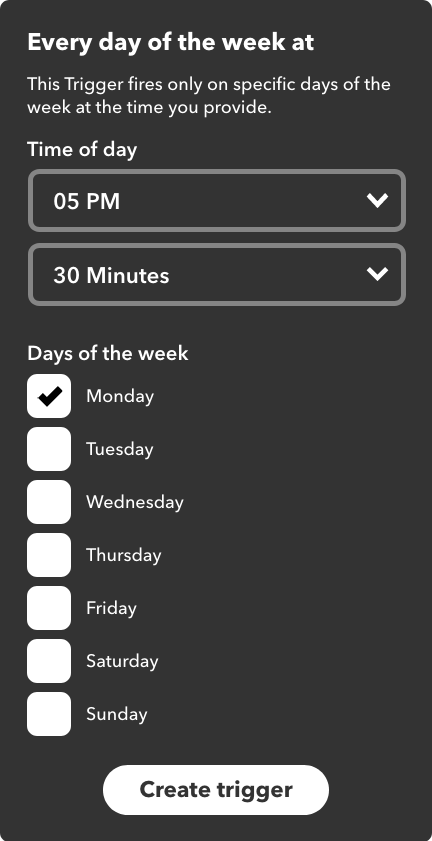The image showcases a scheduling interface designed for a smartphone. At the top, the title "Every Day of the Week at" is prominently displayed in white text against a dark gray background. Directly below, a description reads, "This trigger fires only on specific days of the week at the time you provided." 

The next section specifies the "Time of Day," which is currently set to 5:30 PM. Adjacent to the time setting are white arrows that users can click to adjust the hours and minutes.

Beneath this, a list of days of the week is presented, starting with Monday. Monday has a black checkmark beside it, indicating it is selected, whereas the other days—Tuesday, Wednesday, Thursday, Friday, Saturday, and Sunday—remain unchecked. 

At the bottom of the interface, there is a prominently displayed white button labeled "Clear Trigger." 

The overall layout resembles a typical smartphone screen, suggesting that this user interface is likely designed for mobile use. The dark gray background contrasts with the white text and interactive elements, creating a clean and user-friendly appearance. Several rectangular boxes and customization options populate the interface, supporting user interaction for scheduling and settings adjustments.